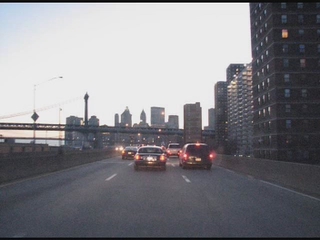This image, likely captured from a dash cam, provides a driver's-eye view from the front of a vehicle traveling down a three-lane road. In the foreground, four cars can be seen ahead, all moving in the same direction on what appears to be an interstate. The vehicles' taillights glow, suggesting that it is either dawn or dusk.

A cityscape stretches across the horizon in the background, characterized by a skyline of diverse buildings. To the right side of the image, additional structures suggest an urban setting. A bridge traverses the photo horizontally about halfway up, leading into the city and becoming partially obscured by the buildings on the right. The sky appears mostly clear with the fading light indicating that twilight is approaching.